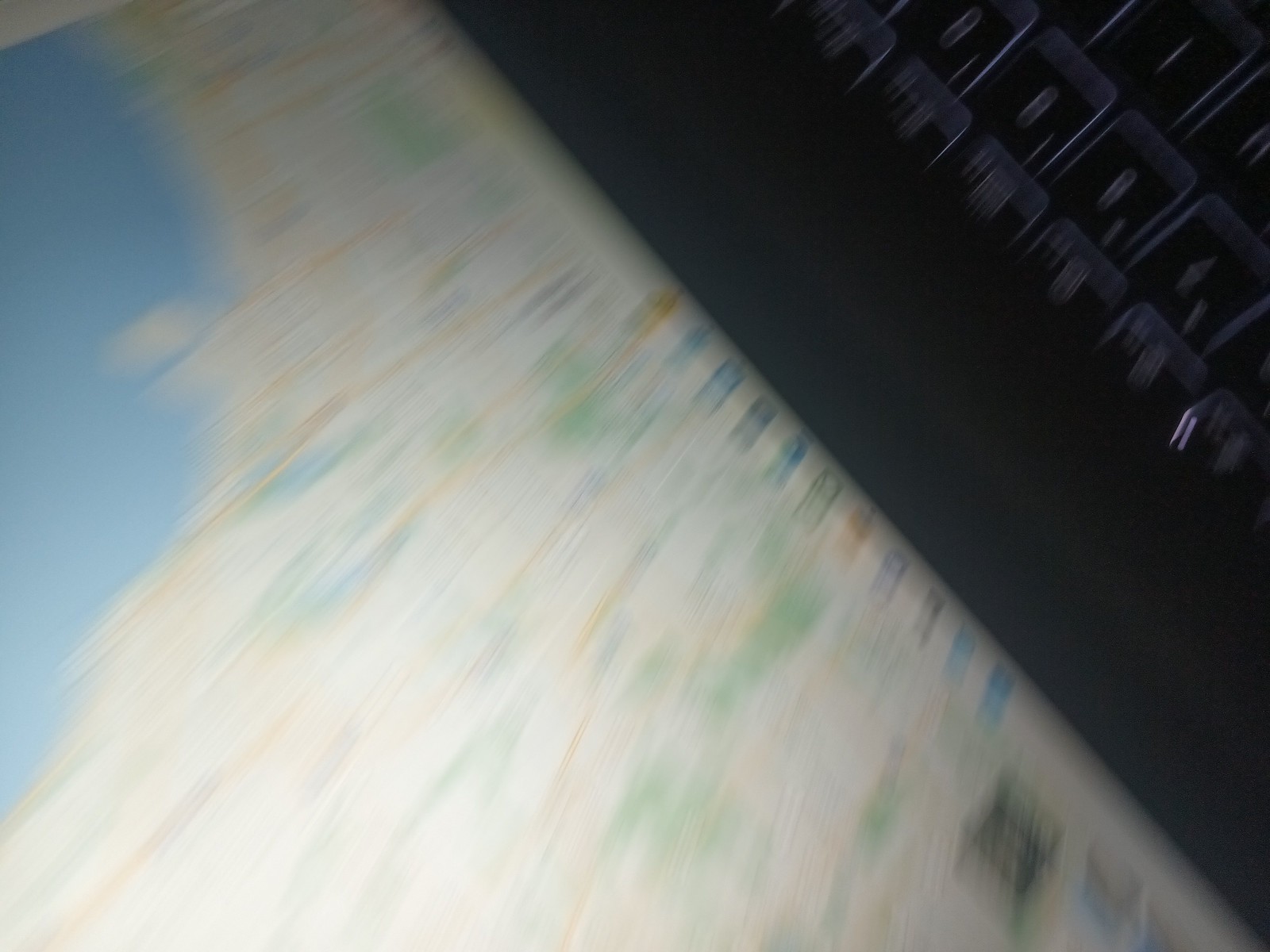The indoor color photograph depicts an upside-down image of a laptop. The screen, occupying the lower two-thirds of the frame, displays a blurred map resembling Google Earth, with indistinct splotches of green, blue, and yellow lines that could indicate parks and roads. The screen is too out-of-focus to reveal specific details or text. A black, backlit keyboard is visible in the upper right corner, with light emanating from around the keys, though individual characters are indistinguishable due to the blur. The distinction between the monitor and the keyboard is marked by a diagonal line stretching from the mid-upper portion of the screen to the lower right. The overall image is highly blurred, rendering the finer details almost impossible to discern but giving a general impression of the laptop and its contents.